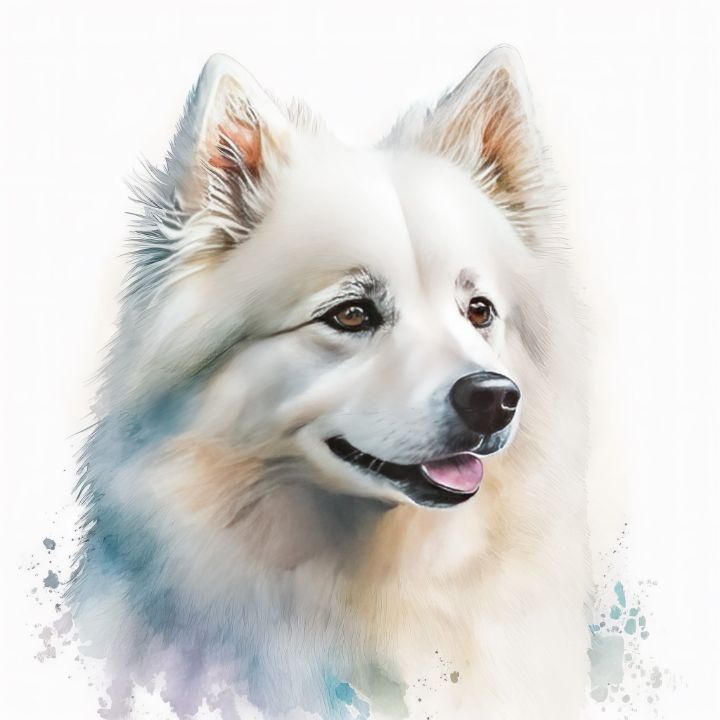This watercolor painting features a striking portrayal of a wolf, or potentially a husky or Samoyed dog, depicted from the neck up against an entirely white background. The animal's face is predominantly white, with a shiny black nose and a partially visible pink tongue that lends an impression of happiness and confidence. Its expressive brown eyes are accentuated with hints of black around them, and its triangular, pointed ears are pink inside, adorned with longer, wispy fur.

The fur texture varies, with the shorter, fluffy fur on its head transitioning to longer, tufted fur as it moves down towards the neck. Light blue shading is skillfully applied under the chin, blending into beige tones around the neck area, suggesting depth and dimension in the fur. Both the bottom left and right corners of the painting showcase light blue, light gray, and some lavender ink splotches, which add artistic flair and contrast to the largely pure upper portion of the artwork. The overall composition beautifully captures the majestic and spirited essence of the wolf or dog, highlighted by subtle yet vivid shading and detailing.